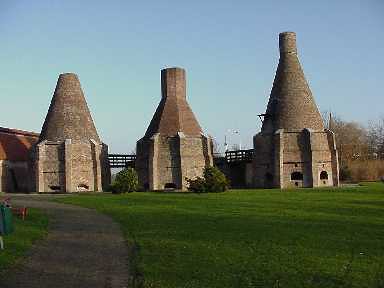The image is a cyan-tinted color photograph taken outdoors in the late afternoon, evident from the long shadows cast by trees over a large grassy lawn at the bottom of the image. Three ancient, stone buildings or towers stand prominently in the center, each with an oddly shaped, somewhat cone-like roof, culminating in either flat tops or narrow vertical chimneys. These structures are constructed from stone and feature small black windows and occasional columns spaced around their circular or multi-sided forms, possibly octagonal. The central building is fronted by small bushes, while a gravel driveway extends from the lower bottom of the image off to the left-hand side, curving as it goes. A small fence is visible behind the buildings, and trees frame the right side of the scene. The photograph appears to be taken from a distance, capturing the architectural details of what might be old furnaces for melting glass, standing resiliently against a cloudless blue sky.